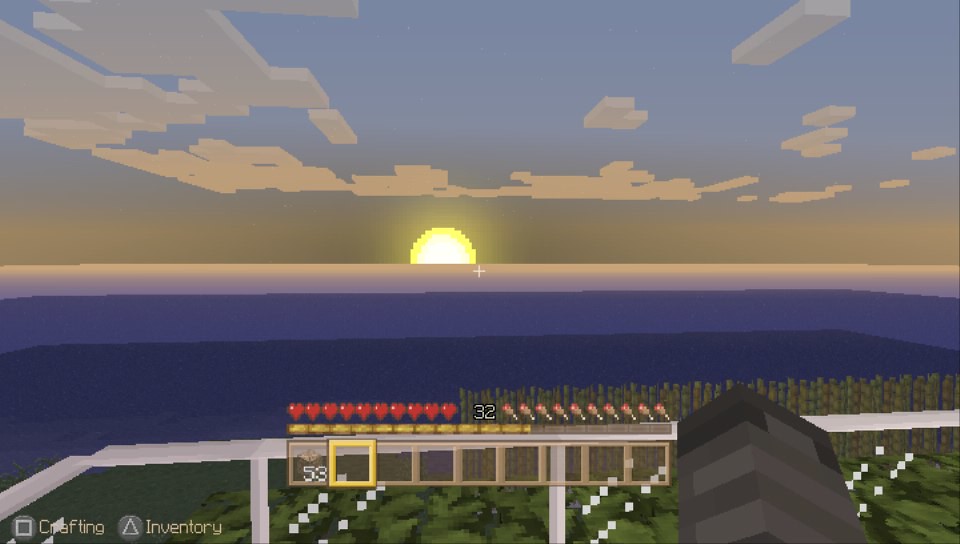This computer-generated image, likely from the game Minecraft, features a distinctive, pixelated environment. The scene displays block-like, rectangular clouds in a square-patterned sky with the sun rising over the horizon. The sunlight brings hints of pink to the sky and reflects off a body of water. At the bottom of the image, a detailed farm area is visible, with what appears to be rows of crops, possibly corn, and patches of green grass or bushes. There's also a game interface overlay: the bottom left shows a square button labeled "crafting" and a triangle button labeled "inventory," representing controller buttons. The player's status bar is filled with heart icons indicating full health and a food inventory count of 32. Additionally, the tip of a Minecraft sword is visible, suggesting the player is ready for action.